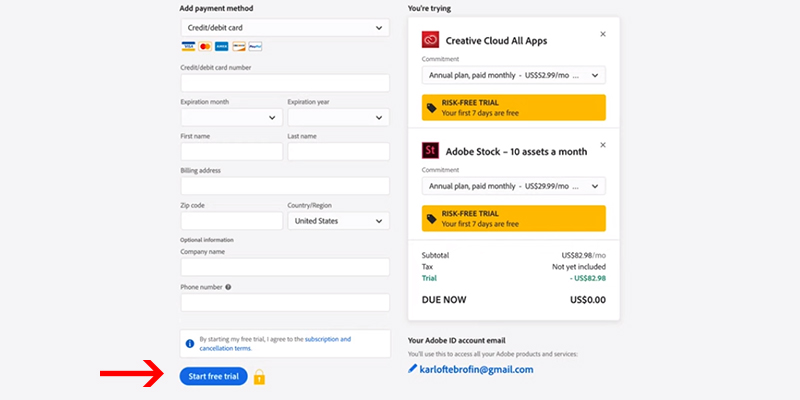The webpage showcases the payment method section prominently at the top with a bolded header "Add Payment Method". Below this header, users have the option to select their preferred payment method from a dropdown menu, which includes options such as credit/debit cards, PayPal, Discover, Amex, MasterCard, and Visa.

Users are prompted to enter their credit card number, expiration month and year (each with individual dropdown boxes), and first and last names. There are also fields for the billing address and ZIP code, and currently, the country/region is set to the United States, although this is editable. Additional optional fields include the company name and phone number, with a question mark icon adjacent to the phone number field for further clarification.

At the bottom of the section, users have to agree to the subscription cancellation terms, which are highlighted in blue, before they can start their free trial by clicking the "Start Free Trial" button, also in blue. A small lock icon is present on the right side, indicating secure processing.

On the left of the screen, there's a prominent red arrow pointing towards the main content area. On the right, above a large white box, the text "You're Trying" is noted. Inside this box, users can view their selected plan, which in this case is "Creative Cloud All Apps." This plan is highlighted with a red icon and is described as an "Annual Plan, Paid Monthly" for $52.99 per month, featuring a seven-day risk-free trial.

Additionally, information about Adobe Stock is provided, offering 10 assets for $29.99 per month, also with a risk-free trial. The current total selected is $82.98 per month, with no tax applied, and the free trial ensures no initial payment is due.